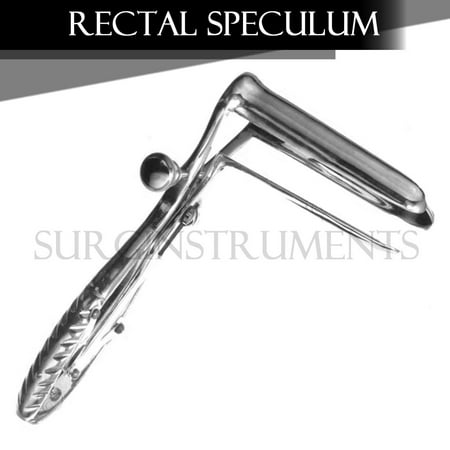The image features a single object, prominently centered against a predominantly white background, which is identifiable as a rectal speculum. This medical tool, primarily silver and chrome in color, is equipped with a sharp, small poker at one end, and features a long handle with indentations for grip. The speculum's design includes a knob near the top, with the handle curving at the tip. The descriptive text "Rectal Speculum" appears in white font on a black banner at the top of the image, while a watermark reading "Surge Instruments" overlays the center of the speculum. The overall setting suggests a clinical environment, such as a doctor's office.